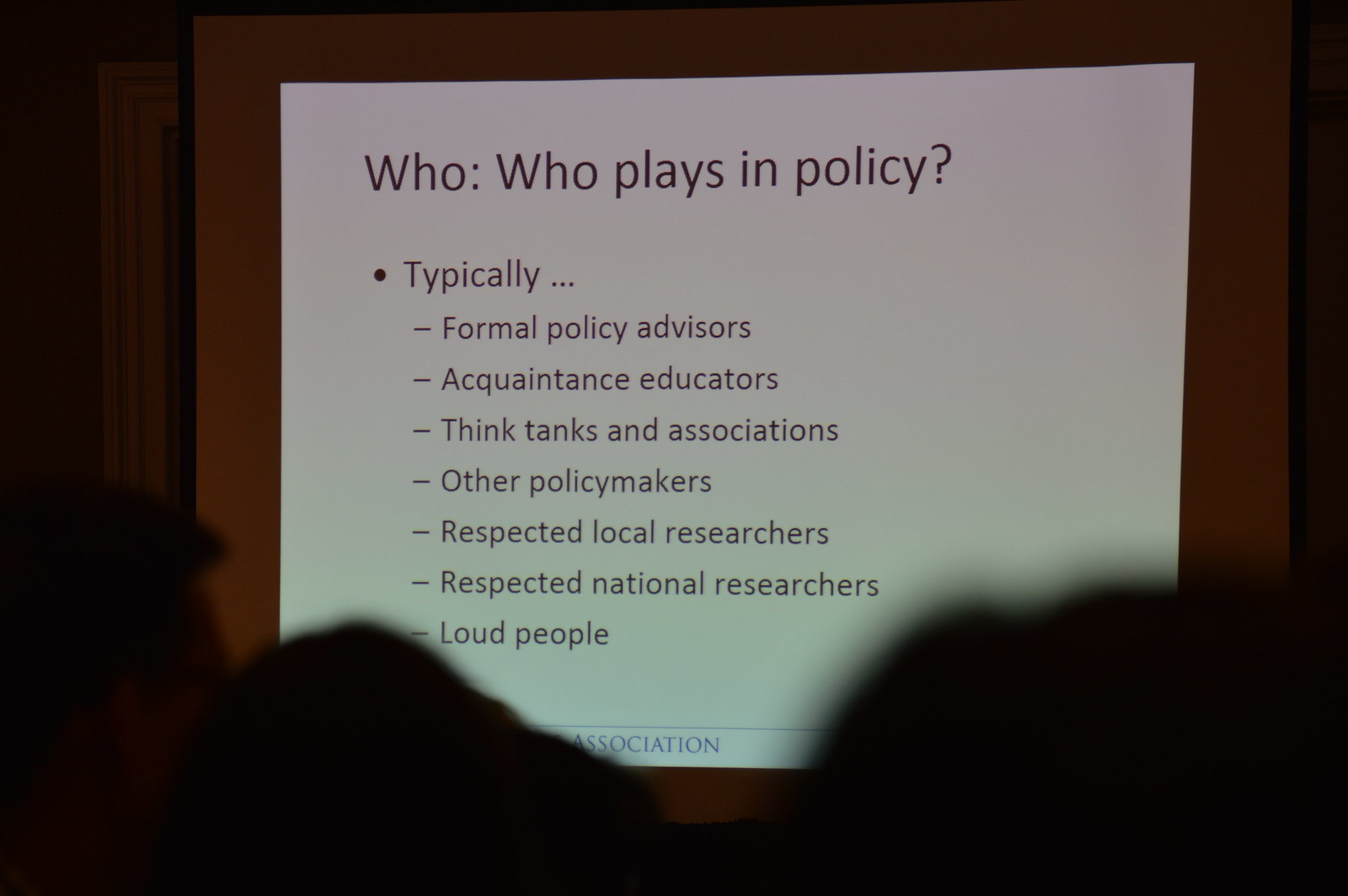The horizontal, rectangular photograph captures a slide projected during a presentation, viewed from the audience's perspective. The main slide, set within a black border, is a white rectangle dominated by text in black ink, devoid of any images or additional background elements. At the top, the bolded title reads “Who? Who Plays in Policy?” Below that, a single bullet point introduces a list that starts with “typically…” followed by the roles: "formal policy advisors, acquaintance educators, think tanks and associations, other policymakers, respected local researchers, respected national researchers, and loud people." The room is dimly lit with an overall dark ambiance, punctuated by a yellowish hue from a single light source. The image also includes the blurred, unfocused heads of attendees at the bottom, some partially obscuring the text on the slide. The slide is slightly off-center against the black background, signifying a typical presentation scene.